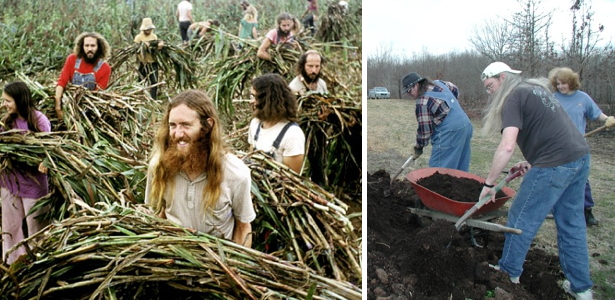This image series features two different settings involving groups of people engaged in outdoor labor. On the left side of the first image, there is a group of at least ten individuals, both men and women, many with long hair, who appear to be working together to gather and carry what looks like cut vegetation or long stalks of dried plants, possibly corn husks or stalks. They are arranged in a loose, circular formation, with some people positioned in the background also taking part in collecting these plants. The attire of the group ranges from white shirts to bib overalls.

In the second image on the right, a more modern scene is depicted showing three people diligently digging in rich, black soil, loading it into a wheelbarrow. The group consists of two men and one woman, dressed casually in attire such as blue jeans, a t-shirt, a flannel shirt, and overalls. Both men are sporting baseball caps, while the woman, standing farther back, also holds a shovel. The setting is an outdoor, grassy area, emphasizing the continuation of communal and agricultural work.